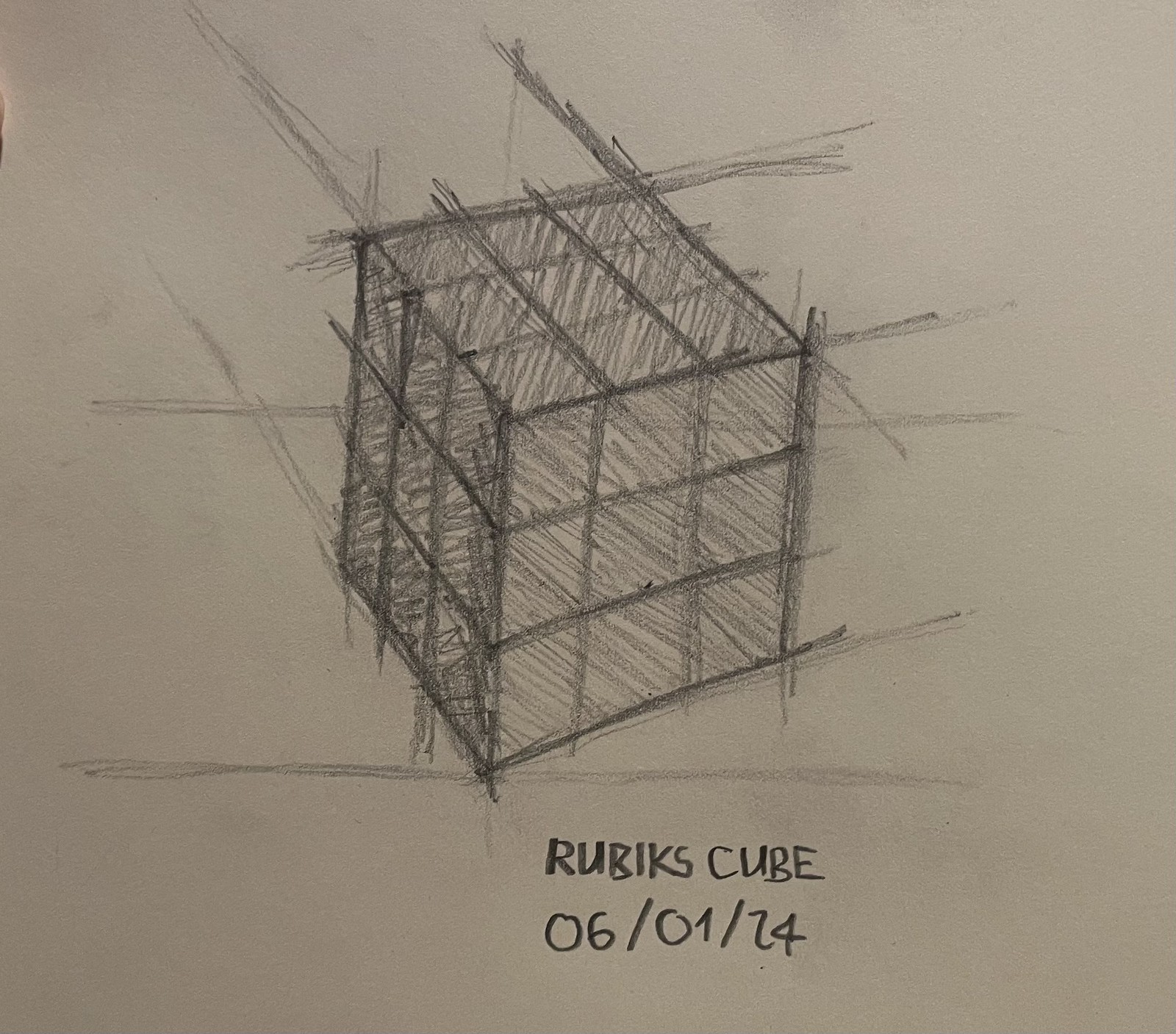The image showcases a detailed pencil drawing on what appears to be a plain white sheet of printer paper or possibly sketch paper. The drawing depicts a cube modeled after a Rubik's cube, complete with smaller squares forming a grid pattern on each face. The bottom of the drawing is labeled "Rubik's Cube 06-01-24" (or possibly "06-01-14"). In the background, faint sketch lines are visible, indicating the artist's efforts to meticulously center and align the cube's elements. Though the illustration lacks color, varying degrees of shading have been employed to distinguish the different sides of the cube.